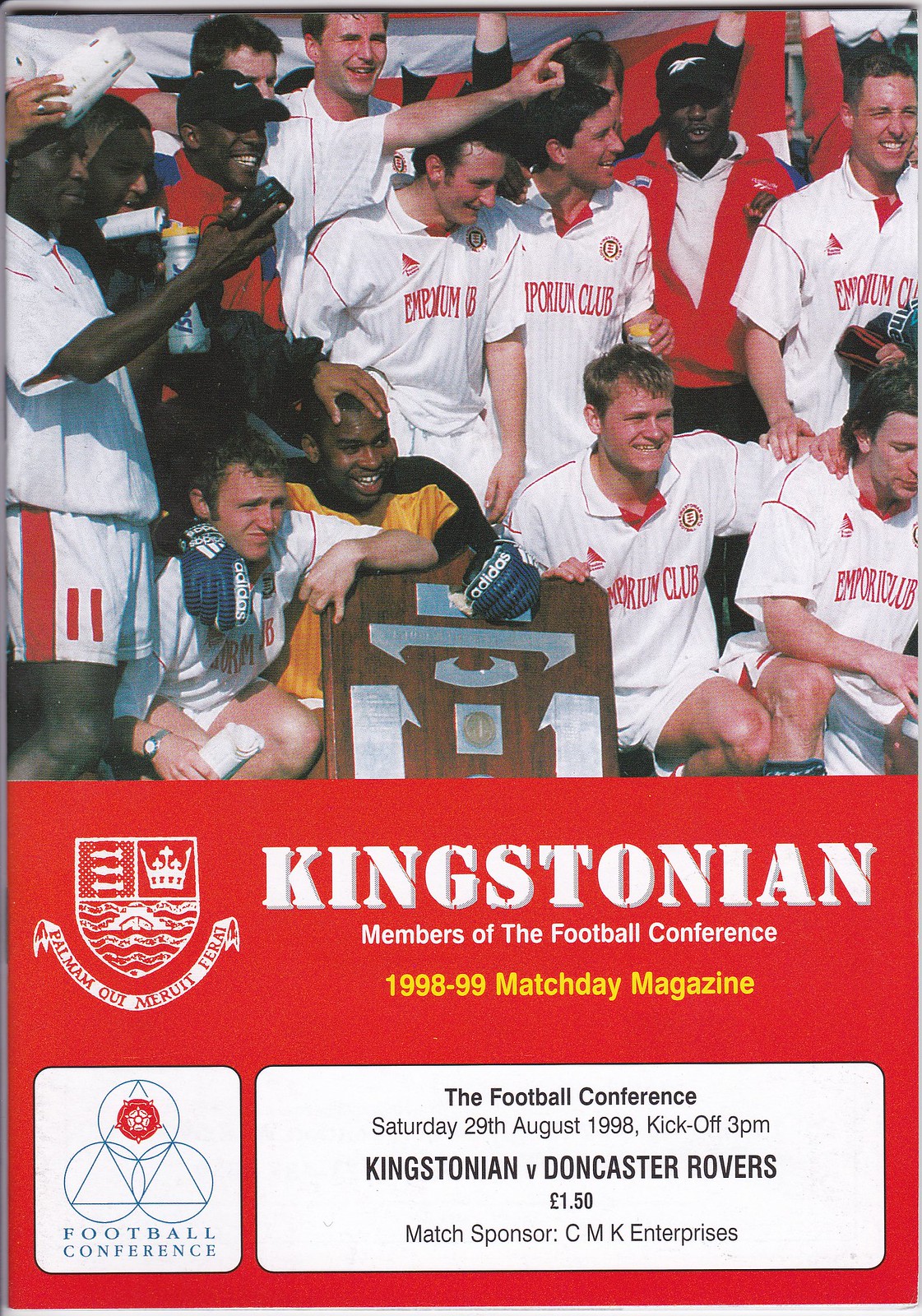The image is a color scan of a match day magazine cover from the football season of 1998-1999, specifically for the Kingstonian Football Club, members of the football conference. The top of the cover features a photograph of the Kingstonian team, comprising players in white uniforms with red lettering and several coaches in red jackets. The players are posed, celebrating and smiling, with a large trophy board visible in the background.

Below the team photo, there's prominently placed text in white font, except for the phrase "1998-99 Match Day Magazine," which is highlighted in yellow. The middle section includes a detailed shield icon adorned with fish, a crown, bars, and a banner inscribed with "Palamautmuritferat." Next to the shield, another text states, "Kingstonian. Members of the Football Conference."

In the bottom left corner, there is a white rectangle containing three triangles with circles inside, labeled "Football Conference." Adjacent to this, in a long white box with black text, details the match specifics: "The Football Conference. Saturday, 29th August 1998, Kickoff 3 p.m. Kingstonian vs. Doncaster Rovers. £1.50." The match sponsor, CMK Enterprises, is also mentioned at the bottom.